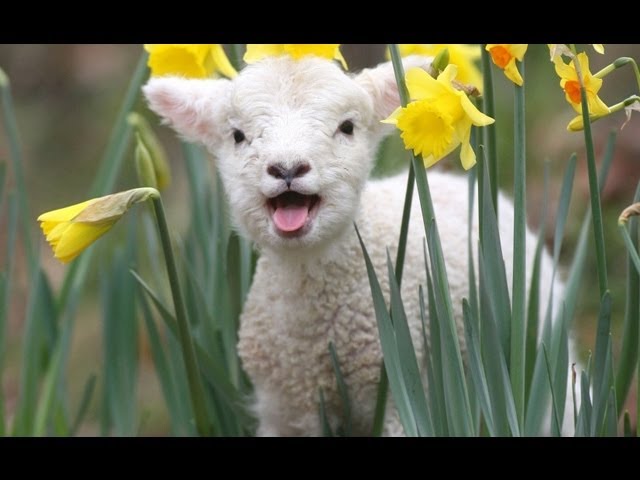In this serene and adorable photograph, a very young white baby lamb with short, curly fur and fluffy legs stands peeking through tall yellow daffodils with some orange centers. The lamb's mouth is slightly open, revealing its pink tongue, giving the impression of a happy, contented expression akin to a smiling dog. Its dark eyes are staring forward, and its black nose and pointed ears, with pale pink insides, add to its charming appearance. The tall green stems of the daffodils surround the lamb, with a few flowers in the background blurring into an artistic fashion. The close-up image captures the peaceful and soothing essence of this cute little lamb amidst the bright and isolated daffodils.